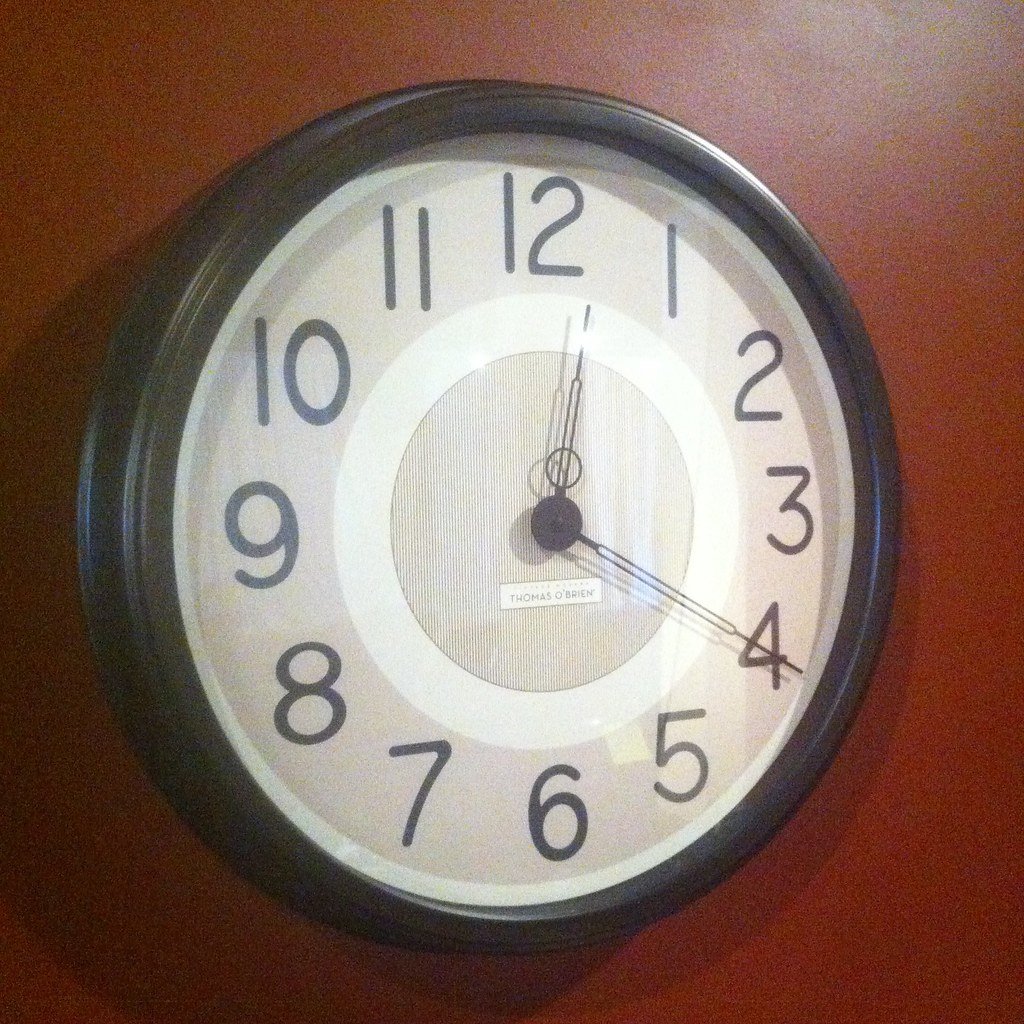The image features a round clock mounted on a dark brown surface. The clock is framed by a black rim and showcases the numbers 1 through 12 in a traditional layout. Encircling these numerals is a white ring, which is itself bordered by a light gray ring that matches the background color for the numbers. At the very center of the clock, a black disc securely holds the hour and minute hands, which indicate the time as 12:20. Notably, there is no second hand present. The centerpiece of the clock face features a rectangular logo that reads "Thomas O'Brien."